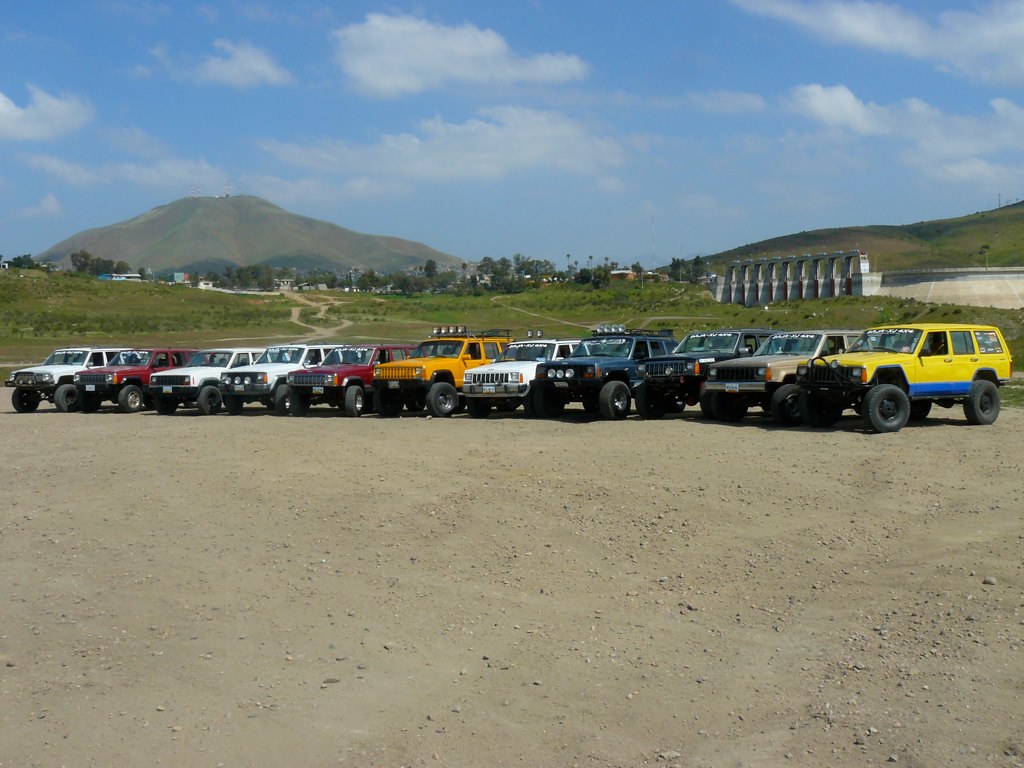This photograph captures a vivid scene of an off-road assembly, featuring a lineup of approximately 11 Jeeps parked in a sprawling dirt lot scattered with patches of gravel. The vehicles, varying in color from yellow, blue, tan, navy, white, orange, to red, suggest a Jeep rally or off-road event, with many sporting oversized tires and lift kits. Surrounding the dirt area is a backdrop of green hills and trees, interspersed with small houses and paths. There are also some ambiguous cement structures to the right side of the image, possibly a bridge or dam. Overhead, the sky is a bright blue, dotted with fluffy white clouds, further enhancing the lively and adventurous atmosphere of the scene.